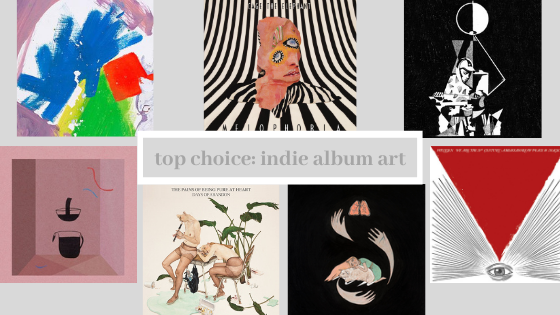The image is a curated collection titled "Top Choice: Indie Album Art," prominently displayed in dark gray text on a lighter gray rectangular header with a white border, centered within the frame. The collection features seven unique illustrations arranged in two rows—three on the top row and four on the bottom.

In the top row, the first piece is a smudgy painting with a vibrant mix of blue, green, red, and yellow hues. Next to it, there is an eye-catching depiction of a two-eyed woman in red, black, and white stripes. The last image on the top row showcases a person working on a chair under a circular object, all set against a black backdrop.

The bottom row starts with an illustration of a coffee cup and coffee machine, with a pink box situated to the right of them. Adjacent to this, an almost naked individual plays the flute next to another figure, with both partially out of frame and a green plant beside them. Following this, there is an image with a black backdrop featuring two cats, surrounded by hands, with a pair of brown lungs positioned above them. The final image in the collection is a striking black and white eye with radiating black and white lines and a red triangle hovering above it.